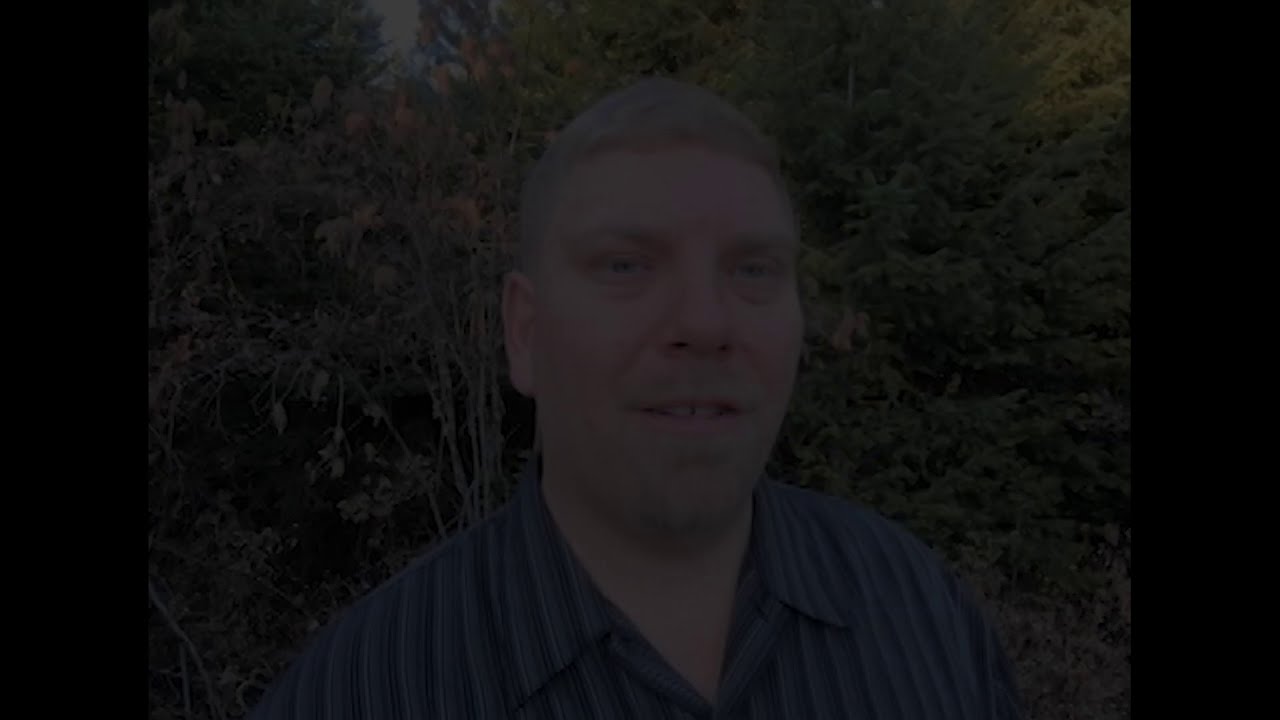This dimly lit photograph captures a Caucasian man, possibly in his mid-40s, standing in front of indistinct green bushes and pine trees. Due to extremely low brightness and heavy contrast, the details are quite obscure. The man has short, light-blonde hair and a very short-cropped beard and mustache. His blue eyes appear tired with noticeable bags under them. He has a straight, full nose and a small gap between his front upper teeth, which are visible as his mouth is slightly open, suggesting he may be mid-speech. He is dressed in a blue button-up collared shirt with horizontal stripes in various shades of blue. The image, seemingly a screen grab, also has black borders on both sides, adding to its peculiar, low-exposure quality.